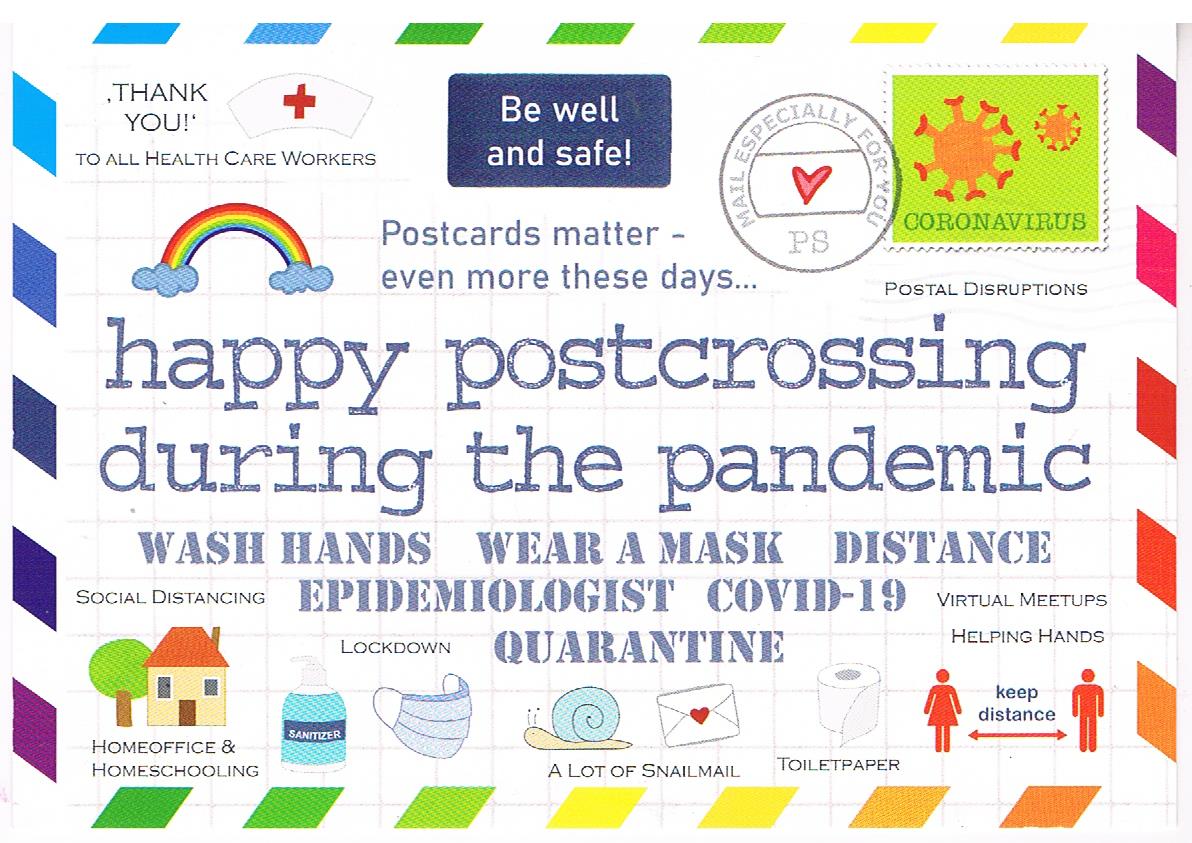The postcard features a vibrant border with slanted rectangles in various colors: green, yellow, red at the bottom; blue, green, yellow at the top; and purple, red, yellow, blue, purple on the sides. At the top center, in a black background, a message reads "Be well, be safe." To the left, it acknowledges the efforts of healthcare workers with "Thank you to all healthcare workers" next to a white nursing hat with a red cross. Beneath it, another note states, "Postcards matter even more these days." 

The central message, "Happy post-crossing during the pandemic," is prominent and is followed by essential health guidelines: "Wash hands, wear a mask, distance, social distancing, epidemiologist, COVID-19 quarantine, virtual meetup, helping hands." Below this, there are illustrations representing life during lockdown, including home office setups, homeschooling scenes, sanitizers, face masks, and an image of a snail symbolizing "a lot of snail mail." Additionally, there is a picture of toilet paper with a reminder to "keep distance," shown by icons of a man and woman with arrows pointing in both directions. 

On the right side of the postcard, a green stamp with the word "Coronavirus" and its symbol is prominently displayed. To its left, a circular stamp reads "Mail specifically for you."

The postcard encapsulates various aspects and challenges during the COVID-19 pandemic, rendered in a visually engaging and colorful manner.